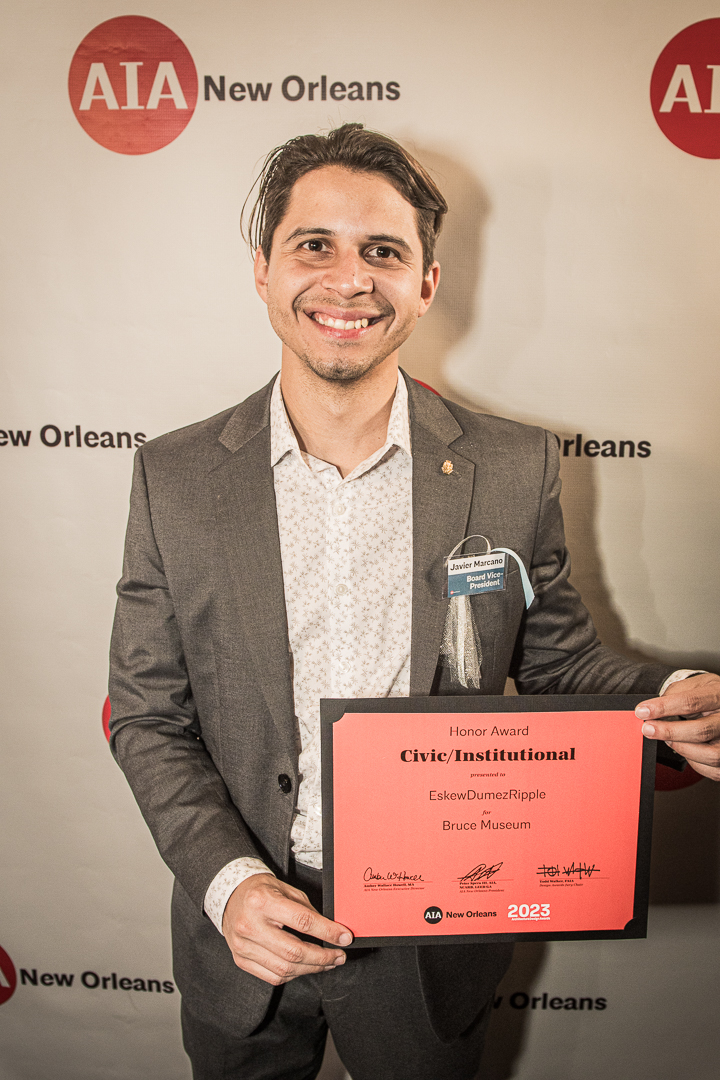In this photograph, a jubilant man with light brown, shoulder-length hair and a broad smile looks directly at the camera, proudly holding up a red certificate in both hands. The man appears to be of Indian descent and has a stubbled beard. He is dressed in a casual brown suit without a tie, paired with a white collared shirt adorned with brown designs, and dark jeans. The background is adorned with a repeating logo featuring white "AIA" text within red circles, along with the words “New Orleans”. The certificate, featuring black text on a red background, announces the "Honor Award Civic Institutional" presented to Eskew Dumas Rippey for the Bruce Museum. The man’s evident happiness seems to mirror the prestigious recognition he has just received.